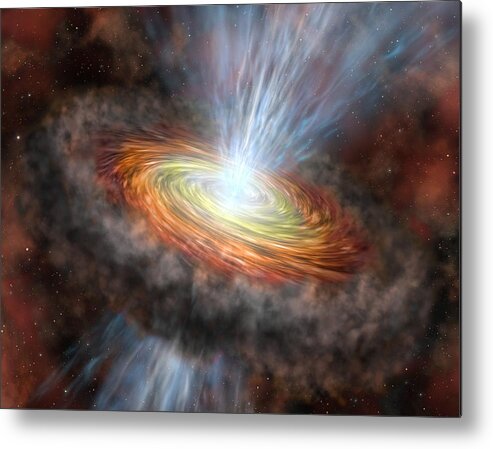This image is a highly detailed, computer-generated or digital illustration depicting a dramatic cosmic event, possibly the formation or explosion of a galaxy or a black hole. The background is a deep black studded with white specks representing stars, creating an expansive space setting. Central to the image is a large, colorful spiral resembling a galaxy, spinning rapidly in a clockwise direction. This spiral exhibits a gradient of fiery colors, transitioning from red and orange on the outer edges through yellow to white at the core.

Perpendicular to the plane of the spiral, a conical stream of bright light and particles, primarily white and blue, is seen penetrating through the center, resembling beams of energy or cosmic jets. This conical stream appears to thread through the galaxy, narrowing as it enters the core and widening as it exits.

Surrounding the vivid central spiral are dark gray and colorful clouds, contributing to the sense of dust and gas swirling around this intense astronomical activity. These clouds include hues of purple and blue, enhancing the dynamic and energetic feel of the scene. The image is set at a slight angle, tilting from the upper left to the lower right, and occupies the majority of the frame, creating an immersive and striking visual experience.